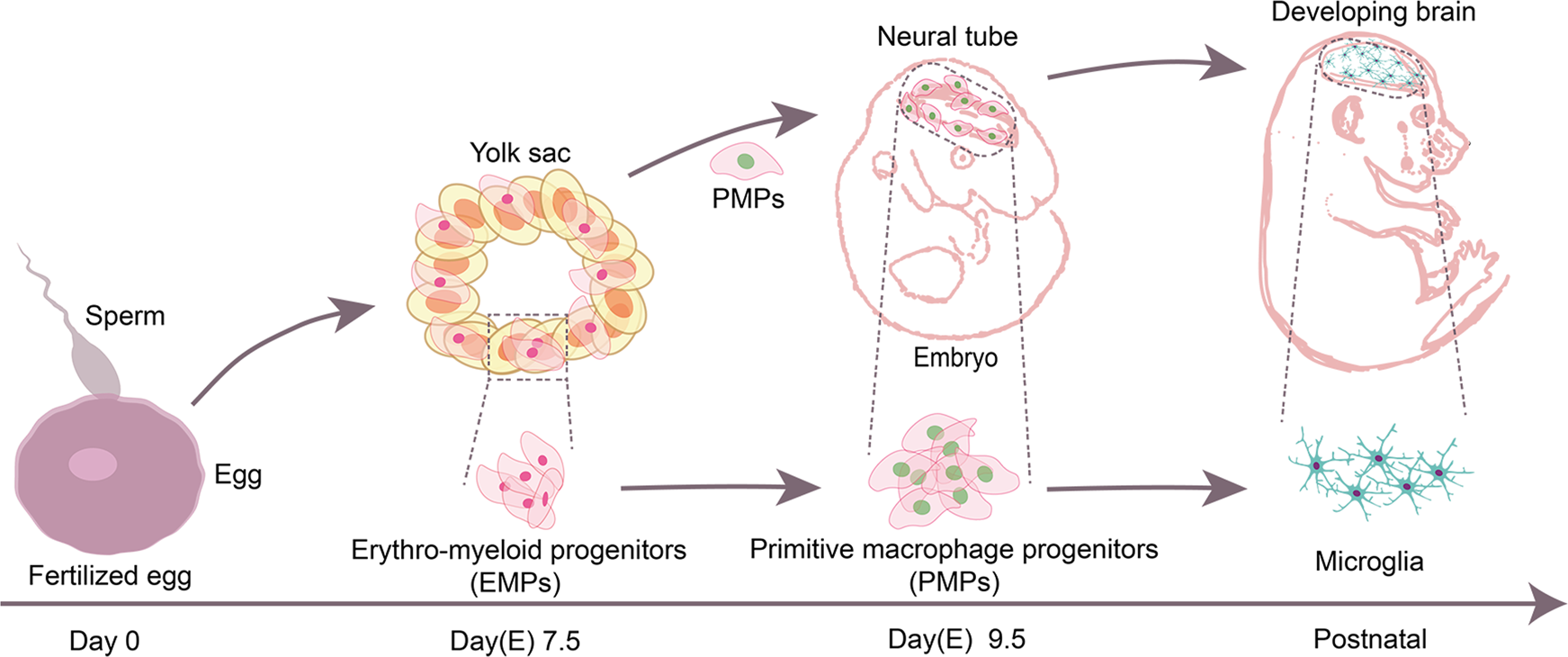This detailed diagram, rich in scientific illustration, depicts the development of a growing animal fetus, likely a dog, across various stages. The timeline is marked by a brownish-magenta arrow pointing to the right, starting from day 0 and progressing through embryonic days 7.5 (e7.5) and 9.5 (e9.5), culminating in a postnatal stage. 

On the far left, day 0, it begins with a depiction of a sperm entering an egg, labeled as "fertilized egg." Moving to day e7.5, the diagram showcases the yolk sac and highlights the presence of erythromyeloid progenitors (EMPs). Another arrow points to day e9.5, where the neural tube is forming, accompanied by an illustration of the embryo, now more distinctly resembling an animal. This stage also notes the presence of primitive macrophage progenitors (PMPs). 

The final illustration shows the embryo with a developing brain, labeled as "developing brain," and indicates the presence of postnatal microglia, subtly capturing the transformation from a fertilized egg to an embryo, and finally to a puppy-like figure with a developing brain. The gradual progression beautifully encapsulates the intricate biological processes at each developmental stage.